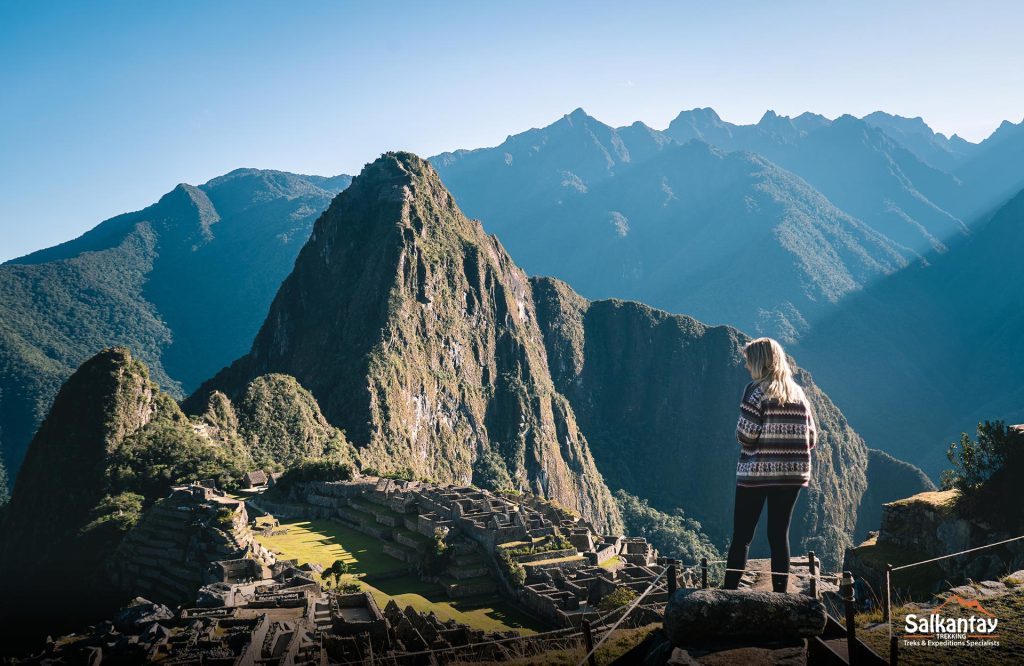A captivating photograph captures a blonde woman from behind, wearing black leggings and a striped white and gray sweater, as she stands at the top of ancient stone steps. She gazes over a vast landscape, dominated by a massive, brown, and seemingly unclimbable mountain that culminates in a sharp apex against a light blue sky. The mountain's sides are adorned with patches of green moss, and its base is dotted with man-made rock gardens and steps leading to various crevices. Other, more approachable hills and flat grassy areas with rope fences serve as guides in the foreground, hinting at a path she might have just ascended or is about to descend. The scene includes more grayish mountains in the background, providing a majestic backdrop to the entire setting. In the bottom right corner, "Salkantay" is printed, accompanied by unreadable smaller text. Neutral tones dominate the image, with refreshing hints of green and yellow.